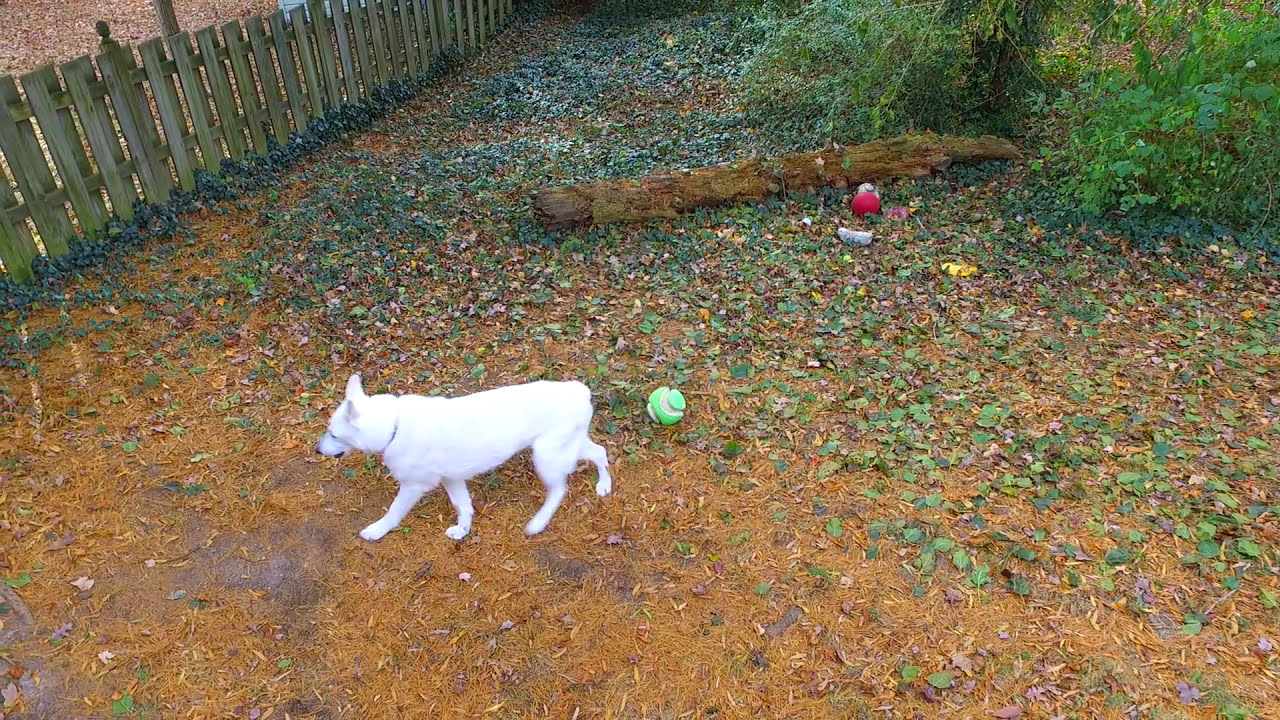The image depicts an overcast backyard, seemingly after a recent rain, indicated by the wet ground scattered with dead leaves, pine straw, and pebbles. A wooden picket fence frames the scene, extending from the left edge, moving diagonally upward to the right, and disappearing out of the frame at the top. Within this fenced-in area, on the top right, there is some green brush. A large fallen tree log lies horizontally in the center of the yard, accompanied by various scattered toys. Near the log, a red and white ball stands out among other indistinct objects. Dominating the middle left of the picture is a medium-sized, all-white dog, comparable in size to a Labrador retriever but of a different breed. The dog, with ears erect and no visible tail, prances towards the wooden fence on the left, sporting a collar. Behind him, a green ball lies on the orangish ground, dotted with dead foliage interspersed with patches of bright green leaves and grass. Additional toys are dispersed further into the yard, contributing to a sense of playful disarray.